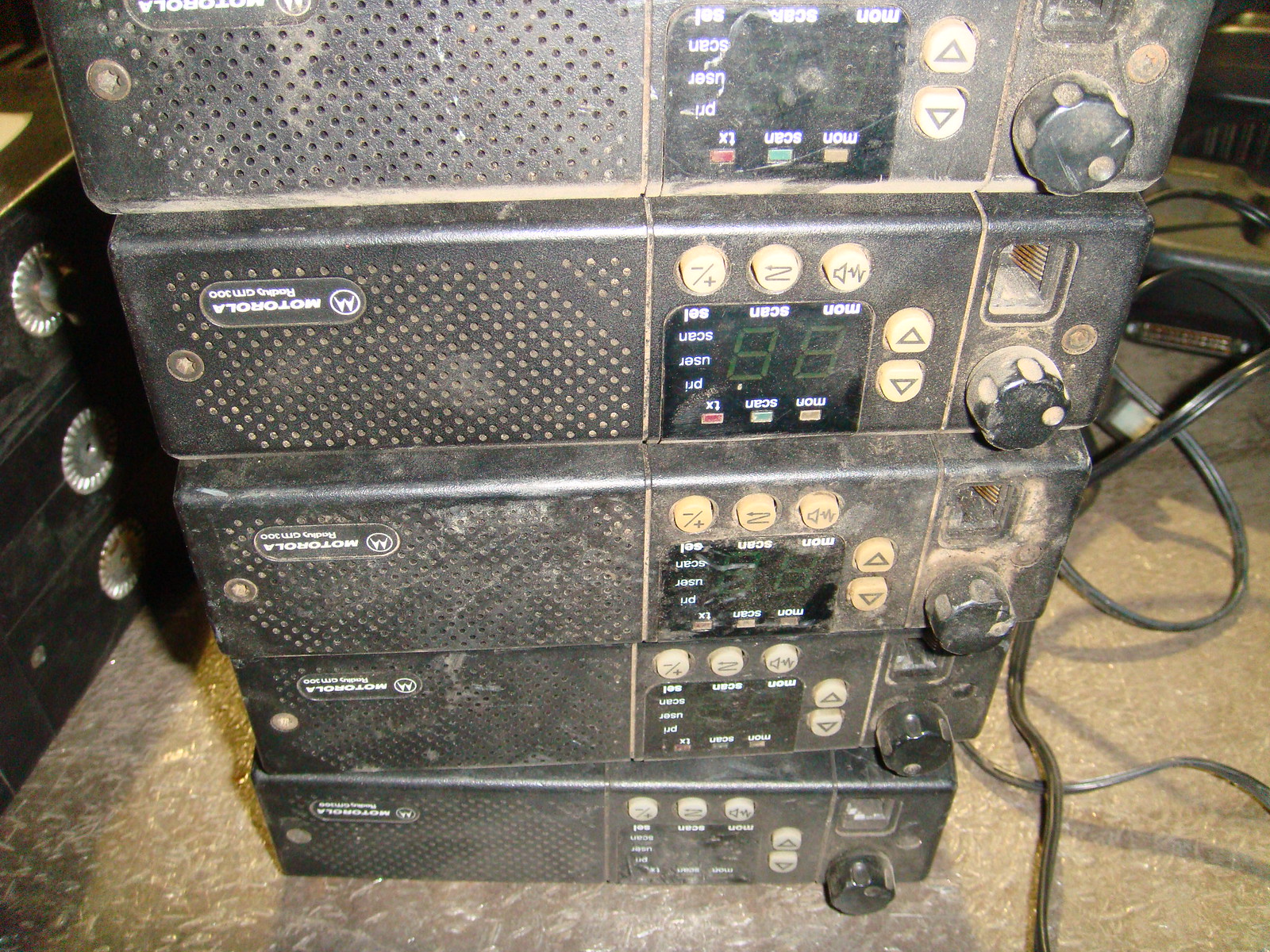This image depicts a stack of five incredibly dusty and dirty Motorola-branded electronic machines, possibly receivers or radios, arranged upside down on an unfinished gray floor. Each machine features a small plastic knob on its right side, with an adjacent arrangement of white and yellow up-down arrow buttons, a mute button, plus and minus buttons, and three yellow buttons adorned with volume symbols. In the middle, a small digital screen can display numbers and various symbols. The left half of each unit has a black speaker-like design, with the upside-down Motorola logo visible at the top left. Black cords extend from these machines, which are accompanied by black drawers or cabinets stacked to their left, and additional indistinguishable, equally dirty equipment to their right.